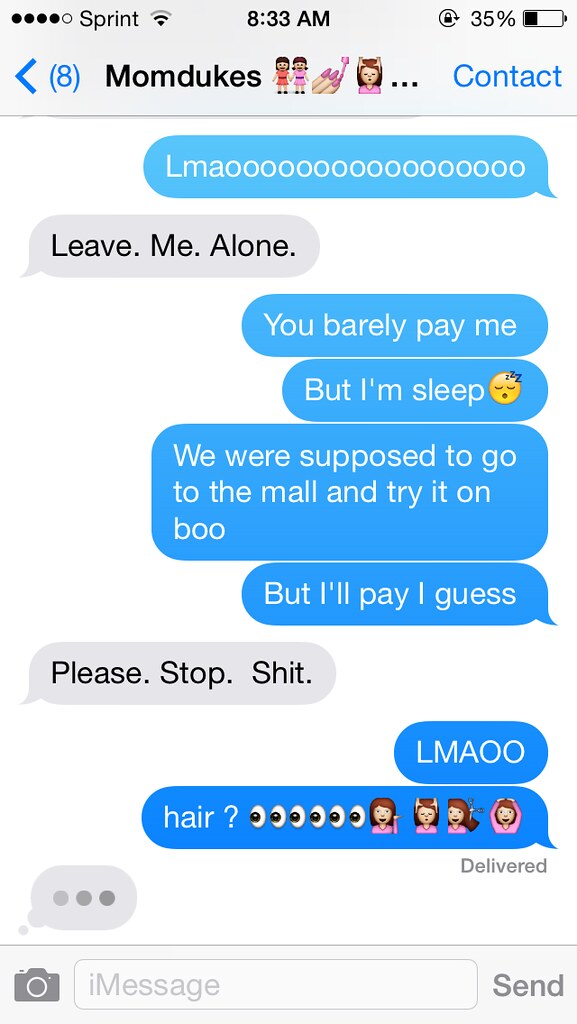This image is a detailed screenshot of an iPhone's text message conversation with a contact named "Mom Dukes," embellished with three emojis: two girls holding hands, nail polish, and a woman carrying something on her head. The top status bar shows that the device is on the Sprint network, connected to Wi-Fi, and it is 8:33 a.m. with the battery at 35%. Additionally, there are eight unread messages indicated.

The conversation unfolds as follows:
1. In blue text, the user sends a lengthy "LMAO."
2. Responding in gray, "Mom Dukes" sternly replies, "Leave. Me. Alone."
3. Four successive messages from the user: 
   - "You barely pay me but I'm asleep" (includes a sleeping emoji).
   - "We were supposed to go to the mall and try it on, boo, but I'll pay, I guess."
4. "Mom Dukes" curtly responds again in gray, "Please. Stop. Shit."
5. The user, in blue, follows up with "LMAO" in all caps and "hair?" with a question mark.

At the bottom of the image, the sending status "Delivered" is visible, along with an ellipsis indicating that "Mom Dukes" is typing a response. The iMessage app interface alludes to a standard iPhone chat setup.